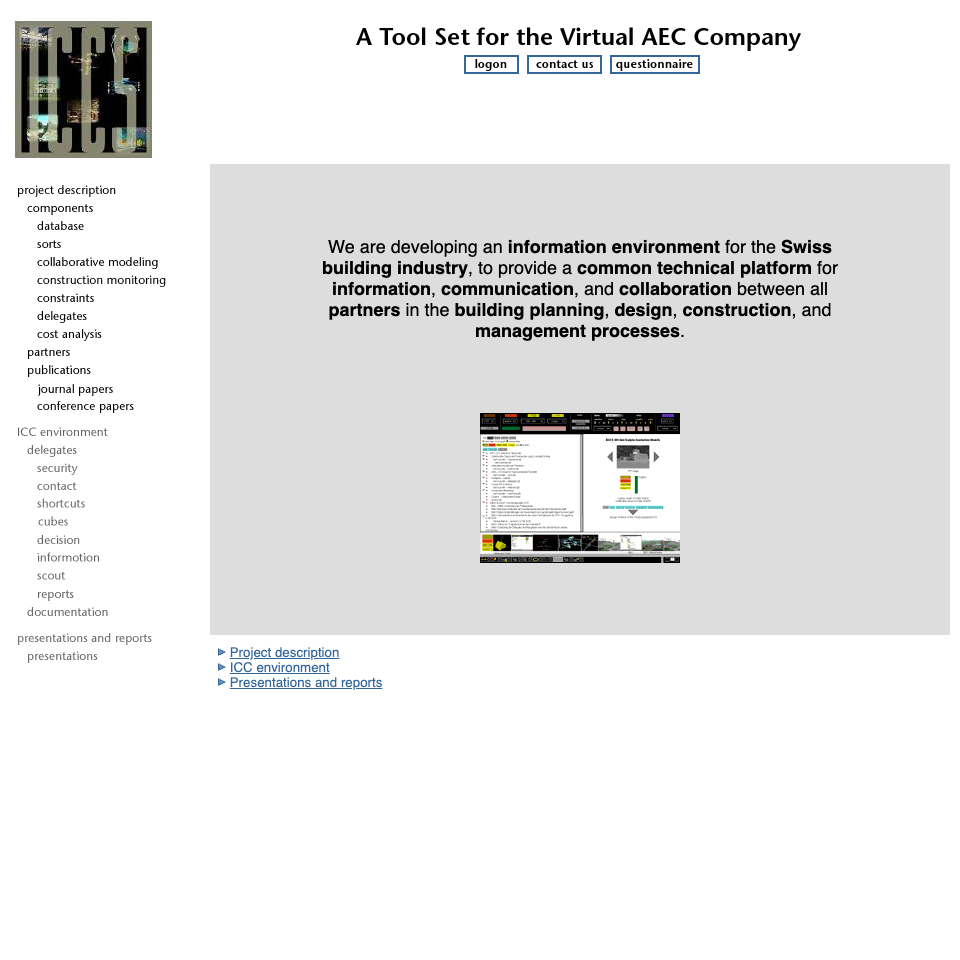This image is a screenshot from an unidentified software interface tailored for the virtual Architecture, Engineering, and Construction (AEC) industry. On its left side, a black square bears the acronym "ICCS," hinting at the overarching system or organization's name. Below this is a comprehensive vertical menu listing numerous functionalities, including: Project Description, Components, Database, Sorts, Collaborative Modeling, Construction Monitoring, Constraints, Delegates, Cost Analysis, Partners, Publications, Journal Papers, Conference Papers, ICC Environment, Delegates again (potential repetition error), Security, Contact, Shortcuts, Cubes, Decision, Information, Scout, Reports, Documentation, Presentations and Reports, and Presentations.

To the right of this menu, a tagline reads: "A Tool Set for the Virtual AEC Company." Below, user options such as Log On, Contact Us, and Questionnaire are available for interaction. A prominent gray square occupies the screen's lower quadrant, containing a message that states: "We are developing an information environment for the Swiss building industry to provide a common technical platform for information, communication, and collaboration between all partners in the building planning, design, construction, and management processes." Key sections highlighted at the bottom of this gray square include Project Description, ICC Environment, and Presentations and Reports.

In the central portion of the screenshot, a sample webpage is visible; however, its details, including text and images, are too small to be discerned. This webpage seems typical of the information and resources users might find within the system.